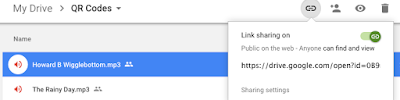The image depicts the user interface of Google Drive, with various elements highlighted and annotated. In the top left corner, the screen displays "My Drive." A dropdown menu is indicated, pointing towards a QR code. On the left side, beneath a name label, the file "howardbwigglebutton.mp3" is listed, identified by a red speaker icon and marked as shared. Below this entry, another file named "thereanyday.mp3" appears, also accompanied by a red speaker icon and marked as shared with people.

A link is present along with icons such as a person, an eyeball, and a gray trash can, denoting sharing settings. The sharing status indicates "Sharable link is on, anyone with the link can view." Further down, a green icon suggests the file is "Public on the web."

Additionally, a URL is provided: "https://drive.google.com/open?id=089," which directs to a specific Google Drive file. The setting tab has text reiterating "My Drive" and "QR code," with the file "howardbwigglebutton.mp3" emphasized. The overall image quality is low, but the annotations and highlighted text are visible, capturing a snapshot of the Google Drive interface with various files and sharing configurations.